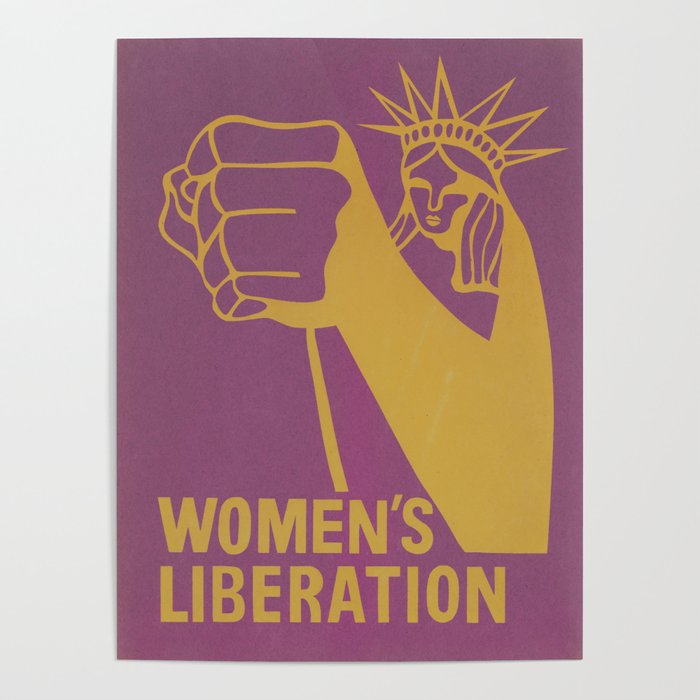The image is a detailed poster set against a white backdrop, featuring the bold and empowering message "Women's Liberation." The words are in gold, all-capital letters with "Women's" on top and "Liberation" beneath it, aligned to the left. The background of the poster is a rich royal purple, symbolizing the importance and royalty of the women's liberation movement. 

Dominating the upper right portion of the poster is a striking gold outline of a female Statue of Liberty. She wears the iconic pointed crown, with long hair cascading down to her shoulders. Her left arm is raised, forming a powerful fist that stretches upward and to the left, symbolizing strength and unity. This image reflects a call for liberation and emphasizes the significant role of women in this movement. 

The combination of the gold illustration and text against the royal purple backdrop makes this poster both visually striking and deeply symbolic.